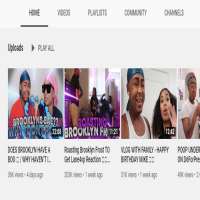Here is a cleaned-up and detailed caption for the image described:

---

This is a detailed screenshot of a YouTube channel's main page. At the top, there is a dark gray navigation banner with several clickable buttons. The first button, labeled "Home", has a black underline indicating it is currently selected. Following "Home", the menu includes "Videos", "Playlist", "Community", and "Changes".

Below this banner, there is a darker gray section featuring bold black text that reads "Uploads", accompanied by a right-pointing arrow, and the words "Play" and "All".

The first video thumbnail in the bottom portion of the screen features a man of African American descent wearing a blue do-rag and a red shirt. Standing next to him is a woman also of African American descent, wearing black sunglasses, a black dress, and a pink do-rag. The video title reads "Does Brooklyn", though the rest is blurred and hard to decipher. The video duration is 13:08.

The next thumbnail shows an individual wielding a violet lightsaber. In the background, there are two individuals also of African American descent, dressed in black clothes and cowering in a corner. The person on the left wears a black shirt and tan pants. The title displayed is "Roasting Brooklyn", followed by "Feet Something". This video's duration is 11:20.

The third thumbnail features an African American man in a sleeveless white shirt and blue do-rag. Accompanying him is an African American woman with curly black hair. The title below indicates "Vlog", and appears to state "Happy Birthday, Make", and "Vlog with Hailey". The video's timestamp is 12:42. On the right-hand side of this thumbnail, the same individual in the white shirt and blue do-rag appears again with what looks like the title "Pop, or Poof Undercover".

---

By refining the initial voice-transcribed text, the caption now provides clear and concise details that accurately describe the contents and layout of the YouTube screenshot.